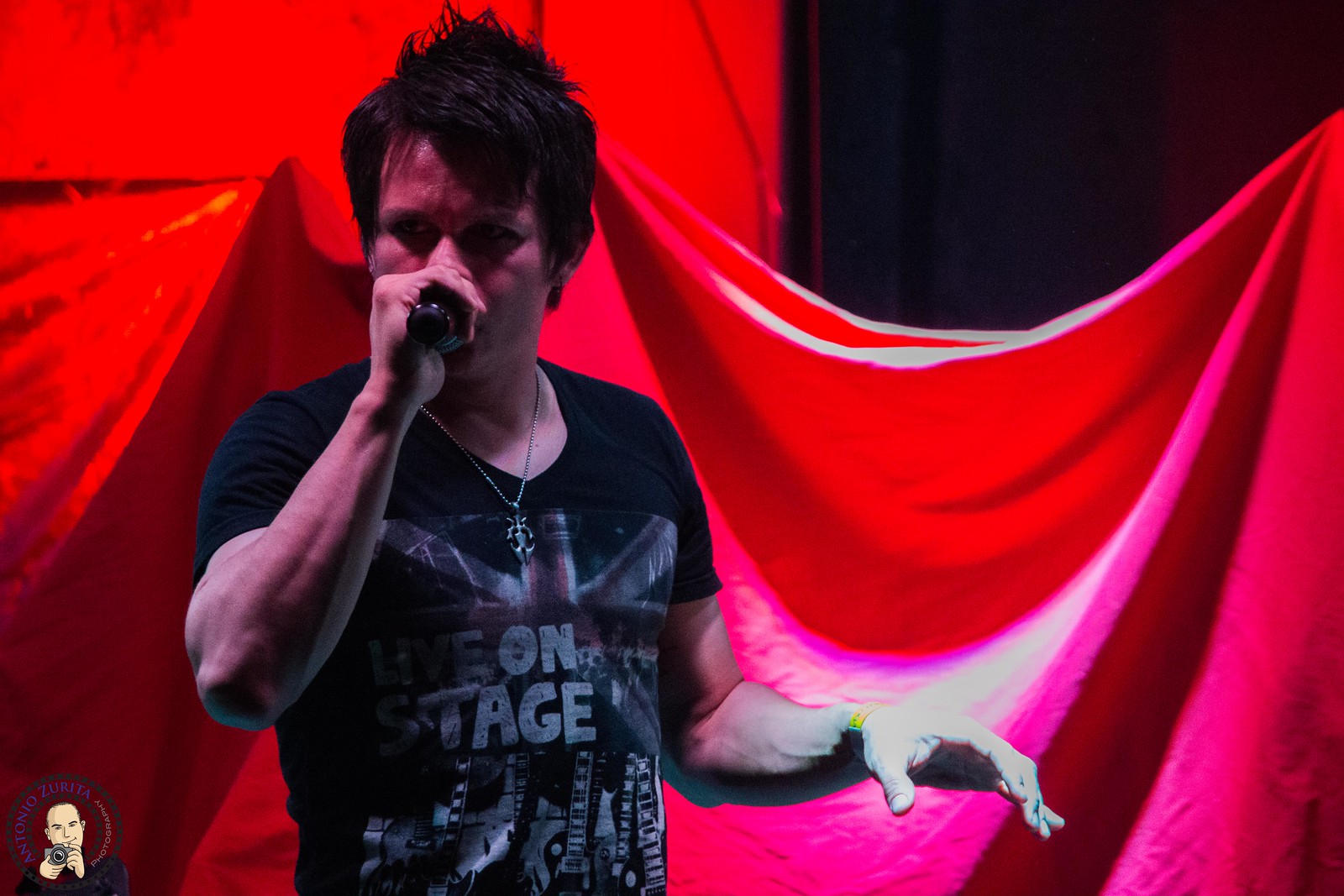The image is a detailed, color photograph in landscape orientation, showcasing a live performance. The central figure is a white man, possibly around 35 years old, with spiky black hair. He stands on the left side of the image, facing the viewer, and holds a black microphone up to his mouth with his right hand, while his left hand hangs by his side. He wears a black t-shirt featuring a faded British Union Jack design and a "Live on Stage" text graphic, possibly with guitars included. A necklace hangs around his neck.

The background consists of red drapery curtains and a combination of a red wall on the left and a black wall on the right. The black wall exhibits various textures from super dark to reddish-tinged dark. In the bottom left corner of the image, there is a small circular graphic depicting a man holding a microphone or camera—likely a watermark or logo reading "Antonio Zurita Photography". The overall setting includes gothic-inspired stage decorations, contributing to the performance's dramatic atmosphere.